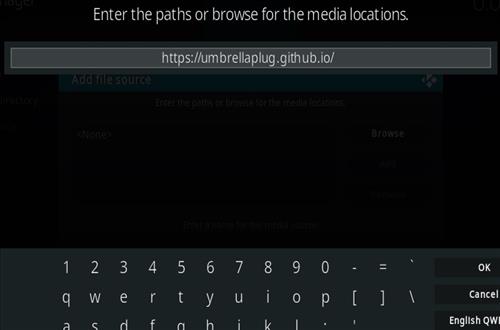The image depicts a pop-up interface on a smartphone screen. At the top of the screen, there is a black rectangular bar with white text displaying the message, "Enter the paths or browse for the media locations." Below this message is a gray input field containing the URL "https://umbrellaplug.github.io/". 

The central portion of the screen is a blank, solid black area, suggesting that no media locations have been entered or selected yet. 

At the bottom of the screen is a detailed QWERTY keyboard layout. The top row of the keyboard includes the numbers 1 through 0, followed by a period, an equal sign, an apostrophe, and an 'OK' button to the far right. 

The next row consists of the letters QWERTYUIOP, with two bracket buttons and a backslash button, concluding with a 'Cancel' button on the right. 

The final row displayed contains the letters ASDFGHJKL, a period, and to the far right, a button labeled "English QWERTY."